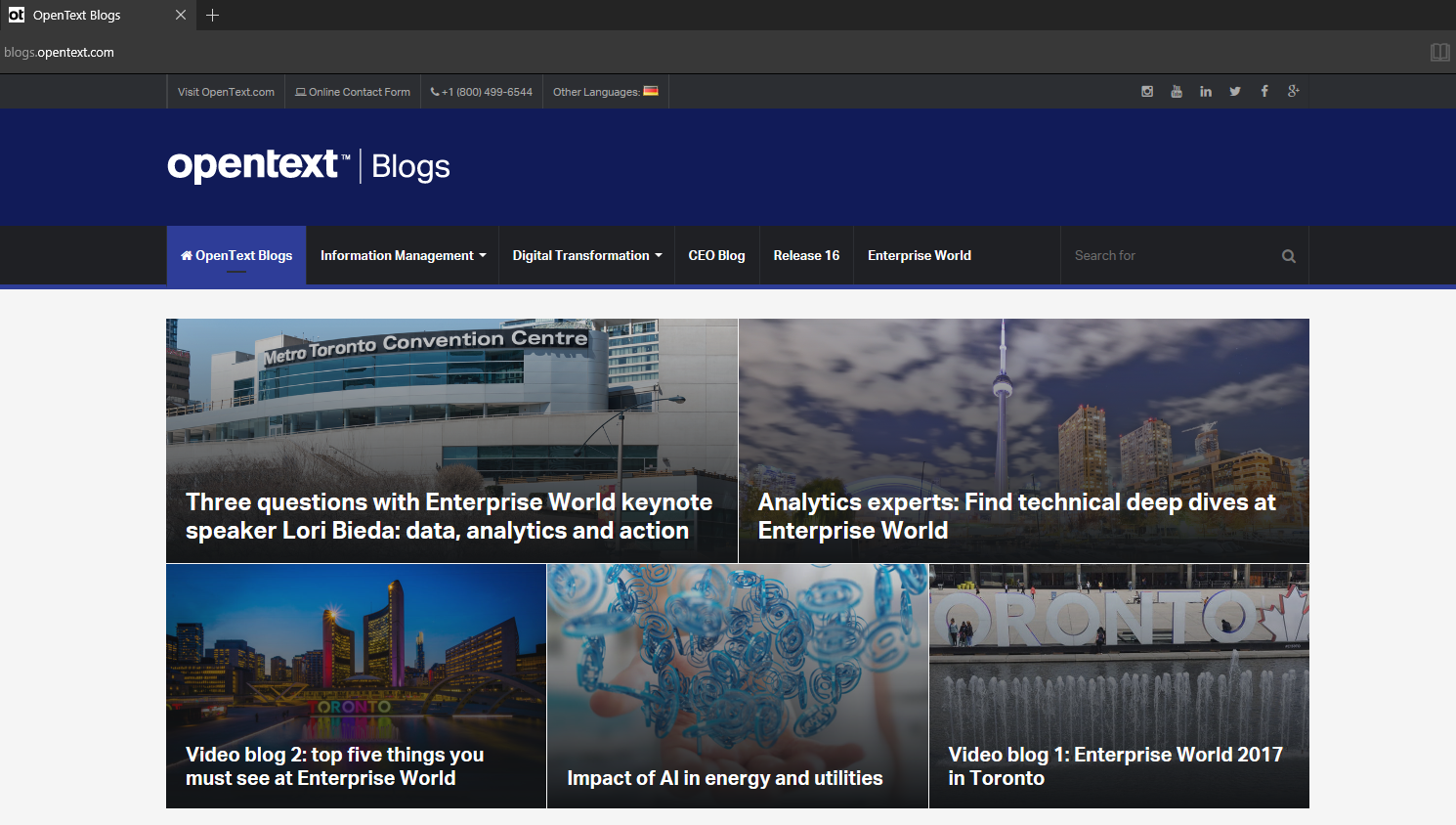In this image, we see a screenshot of the OpenText Blogs website, accessible at blogs.opentext.com. The site's header, located in the upper left corner, prominently displays "OpenText Blogs." Below the header, the web address provided leads to visitopentest.com, with an online contact form and a listed phone number: +1-800-499-6544. Additionally, there is an option to select other languages.

A dark blue rectangular banner on the left features white text that reads "OpenText Blogs." Underneath this banner, there are various navigation tabs, with the "OpenText Blogs" tab currently selected. Other tabs include "Information Management," "Digital Transformation," "CEO Blog," "Release 16," and "Enterprise World." To the right of these tabs is a search bar.

The webpage displays a series of articles, beginning with "Three Questions with Enterprise World Keynote Speaker Lori Beda," followed by "Data Analytics in Action: Analytics Experts Find Technical Deep Dives into the Enterprise World." Another highlighted article is a video blog titled "Video Blog 1: Enterprise World 2017 in Toronto." The layout and organization present a professional and user-friendly interface for readers interested in the latest insights and updates from OpenText.